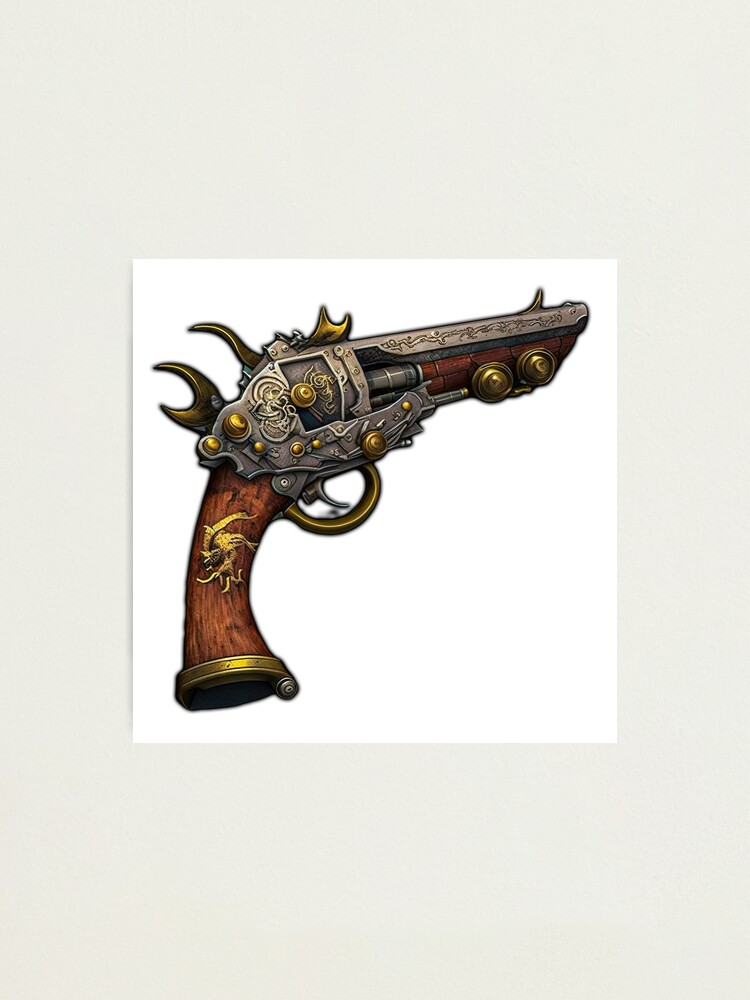The image showcases a detailed, steampunk-style artistic rendition of a six-shooter revolver, set against a gray background in portrait mode. The central focus is a white square that prominently displays the handgun. The revolver features a dark brown wooden handle with an ornate, yellow-gold metal band around its base. An intricate gold emblem, possibly depicting an animal like a horse, adorns the handle. The barrel is a striking combination of silver and gold, with numerous gold dots embellishing the sides. The silver metal on the barrel has a distinctive wavy, tentacle-like design, giving it an almost fantastical appearance. The trigger is uniquely shaped, resembling a tentacle or dragon-like claw. The overall design exudes a vintage, pirate-like aura, yet it appears modern and likely created by AI.